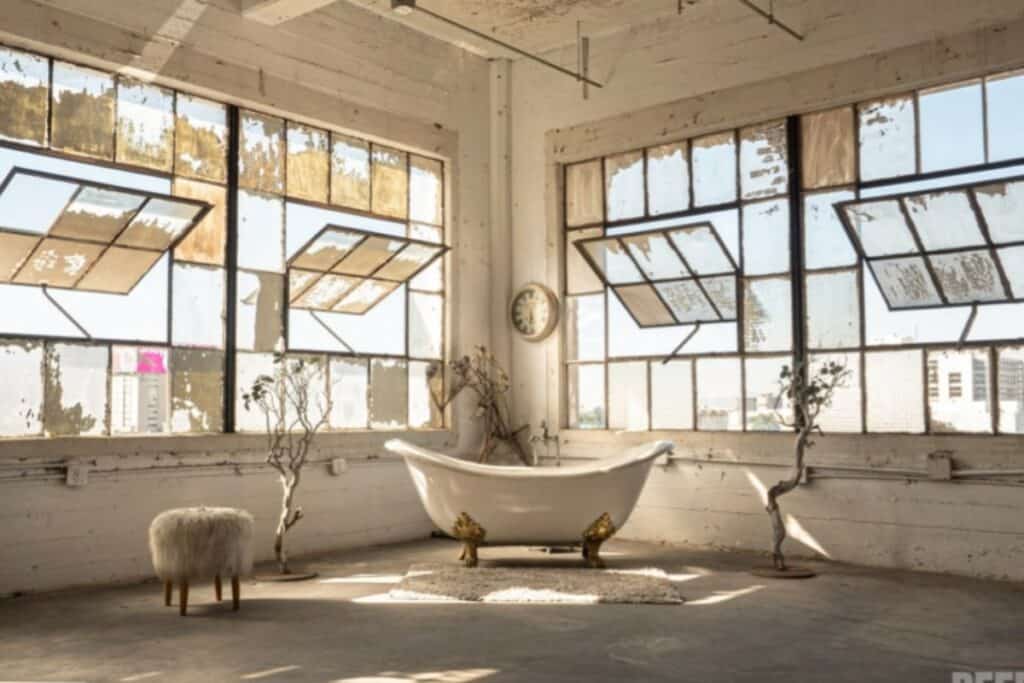This color photograph captures the corner of an urban loft space with a unique blend of rustic farmhouse and industrial aesthetics. The room features white-painted wood floors and ceiling, complemented by almost floor-to-ceiling warehouse-style windows with glass panels that open outward. These large, slightly worn and dirty windows offer a view of green trees, a blue sky, and a faint glimpse of other buildings, including one with a bright pink roof.

Anchoring the corner of the room is a pristine white bathtub with ornate gold claw feet. The bathtub is flanked by two tall, thin decorative trees with very few leaves, giving the space an airy and minimalistic vibe. To the left of the bathtub sits a small, fuzzy stool with a mohair cover, adding a touch of texture and warmth to the space. A clock adorns the wall above, its once-bright surface now dulled by dirt, further enhancing the room's vintage charm. The overall atmosphere is a harmonious mix of natural light, rustic details, and urban elements.